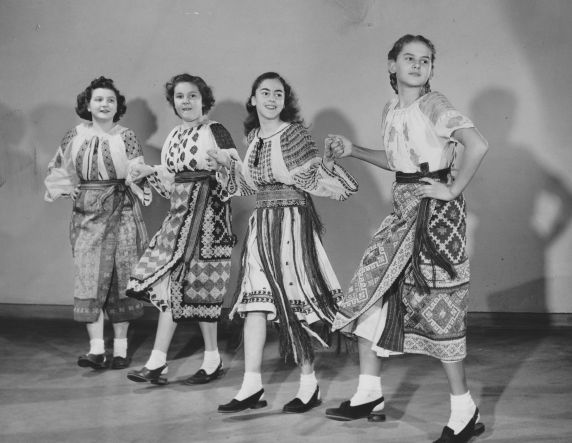A black-and-white photograph captures a joyous moment mid-dance, featuring four young girls, aged around 12 or 13, dressed in traditional garments that appear to be of Mexican, Central, or possibly Latin American origin. The girls, standing in a decent-sized room with a hard floor, are holding hands and smiling as they look off to the right. Each girl wears black dancing shoes and white socks, continuing with long, flowing single-piece dresses. The dresses are white on the top, transitioning into intricate, darker patterns towards the bottom, resembling a patchwork of quilts and threads. The tallest girl on the right has short, dark hair, with her right hand interlocked with the girl beside her and her left hand resting on her hip. The interlocking continues with the second and third girls, while the fourth girl holds the third girl's hand with her right hand by her side. Their joyous expressions are captured in motion, with shadows cast against the wall behind them, adding depth to the lively scene.